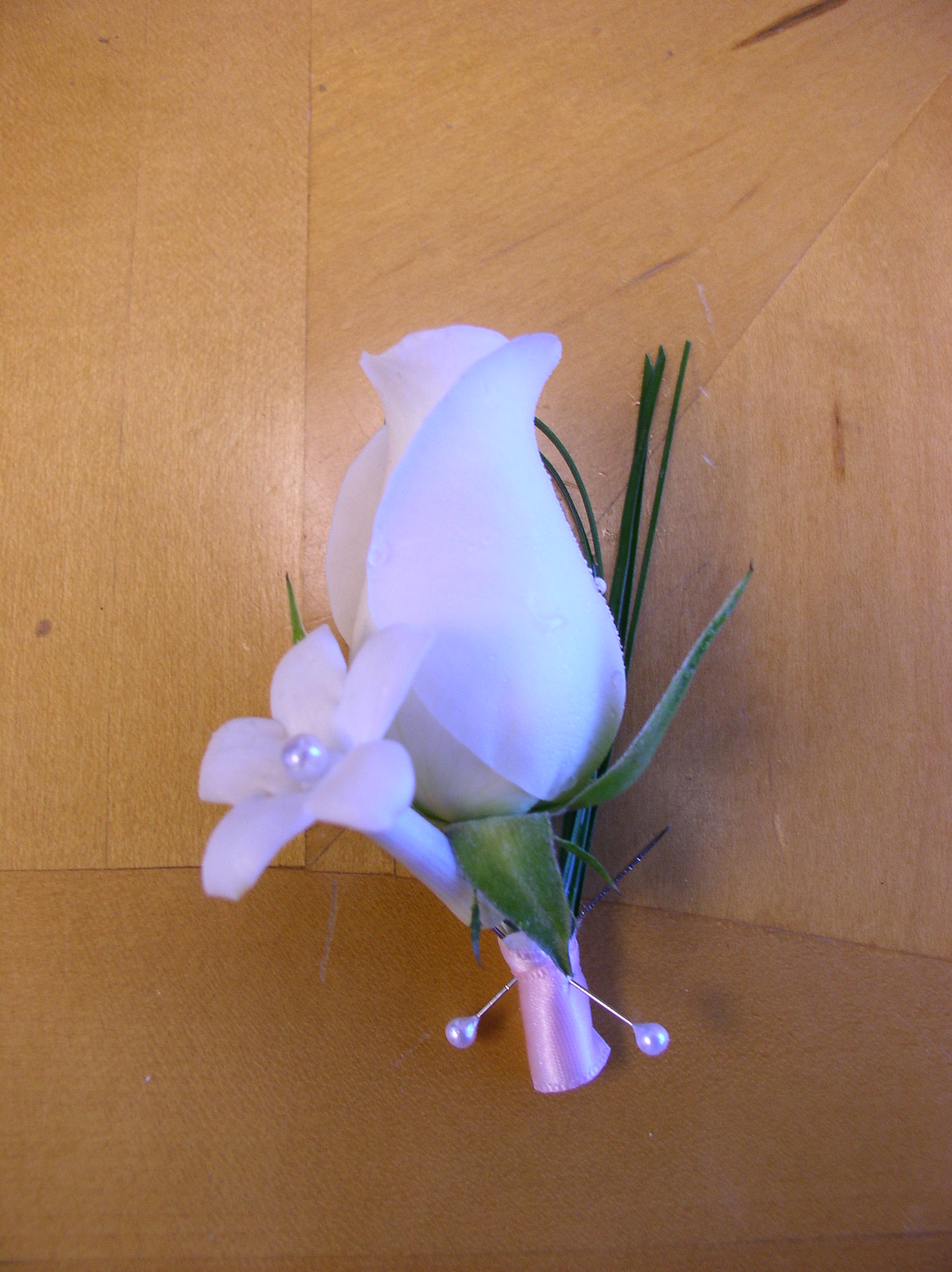This photograph showcases a detailed and elegant boutonniere, designed for placement on a jacket lapel. The focal point is a light purplish or white rose, paired harmoniously with a white daisy-like flower. Each bloom is accentuated by lush, green leaves and sprigs that add depth to the arrangement. A light purple ribbon is meticulously wrapped around the stems of the flowers, holding them securely together. The boutonniere is adorned with two pearl-tipped pins, which are not only functional but also add a touch of refinement. These pins, one of which intriguingly mimics the daisy's pearl-like center, ensure the boutonniere remains in place when fastened to the jacket. The background of the image is a light brown wooden surface, providing a warm contrast to the cool tones of the flowers and ribbon.